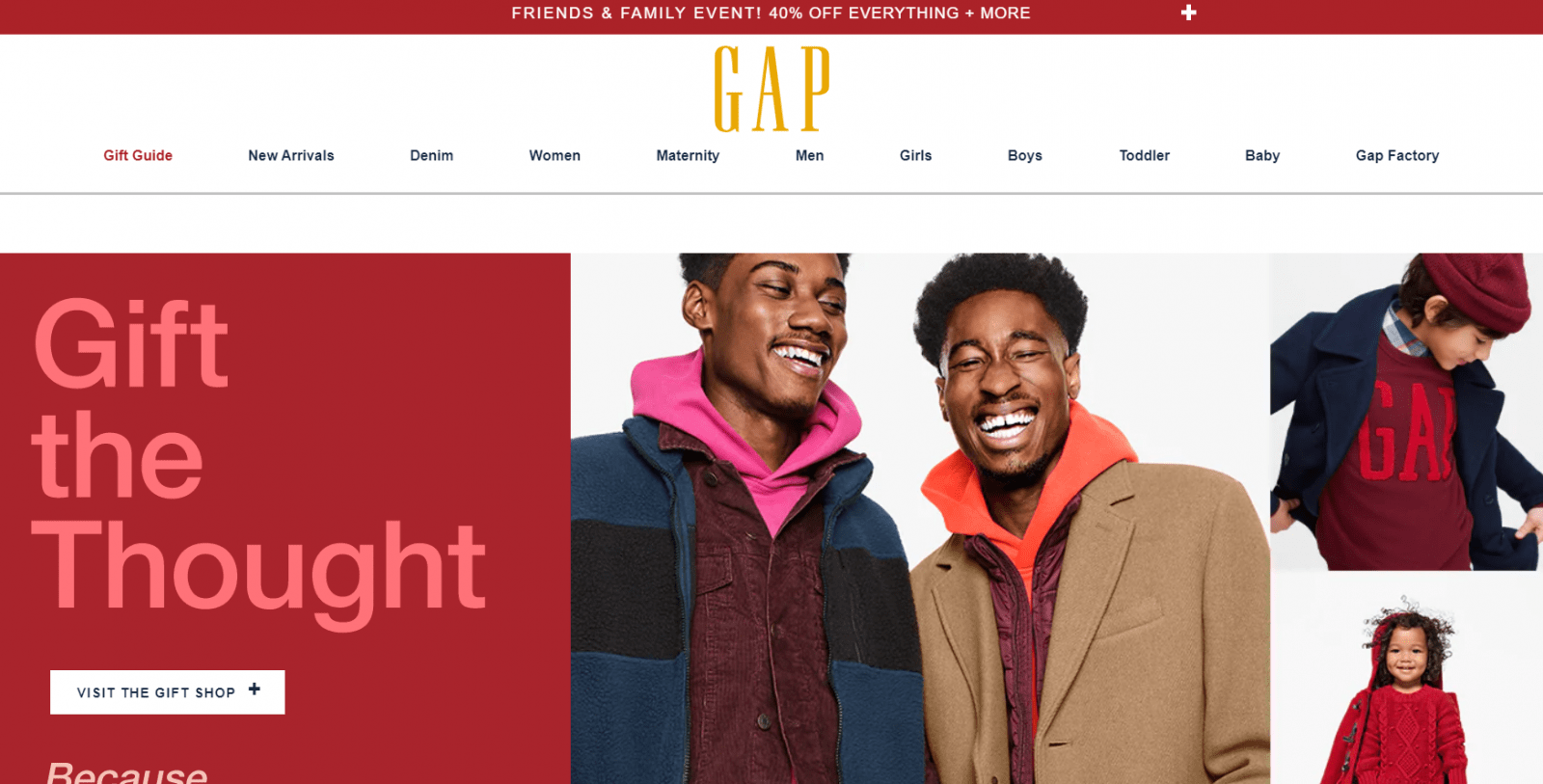The image is a screenshot from the Gap website featuring a promotional banner at the top. The maroon banner announces a "Friends and Family Event" with a highlight of "40% off everything plus more" in prominent white text. Below this, the iconic Gap logo is displayed in gold. The navigation bar features various tabs including "Gift Guide," "New Arrivals," "Denim," "Women," "Maternity," "Men," "Girls," "Boys," "Toddler," "Baby," and "Gap Factory."

On the left side of the image, there is a red box with the phrase "Give Thoughtfully" written in soft pink. Beneath this, a white box with a black plus sign in the corner invites users to "Visit the Gift Shop." The overall layout of the website is clean and user-friendly, highlighting seasonal events and shopping categories for easy navigation.